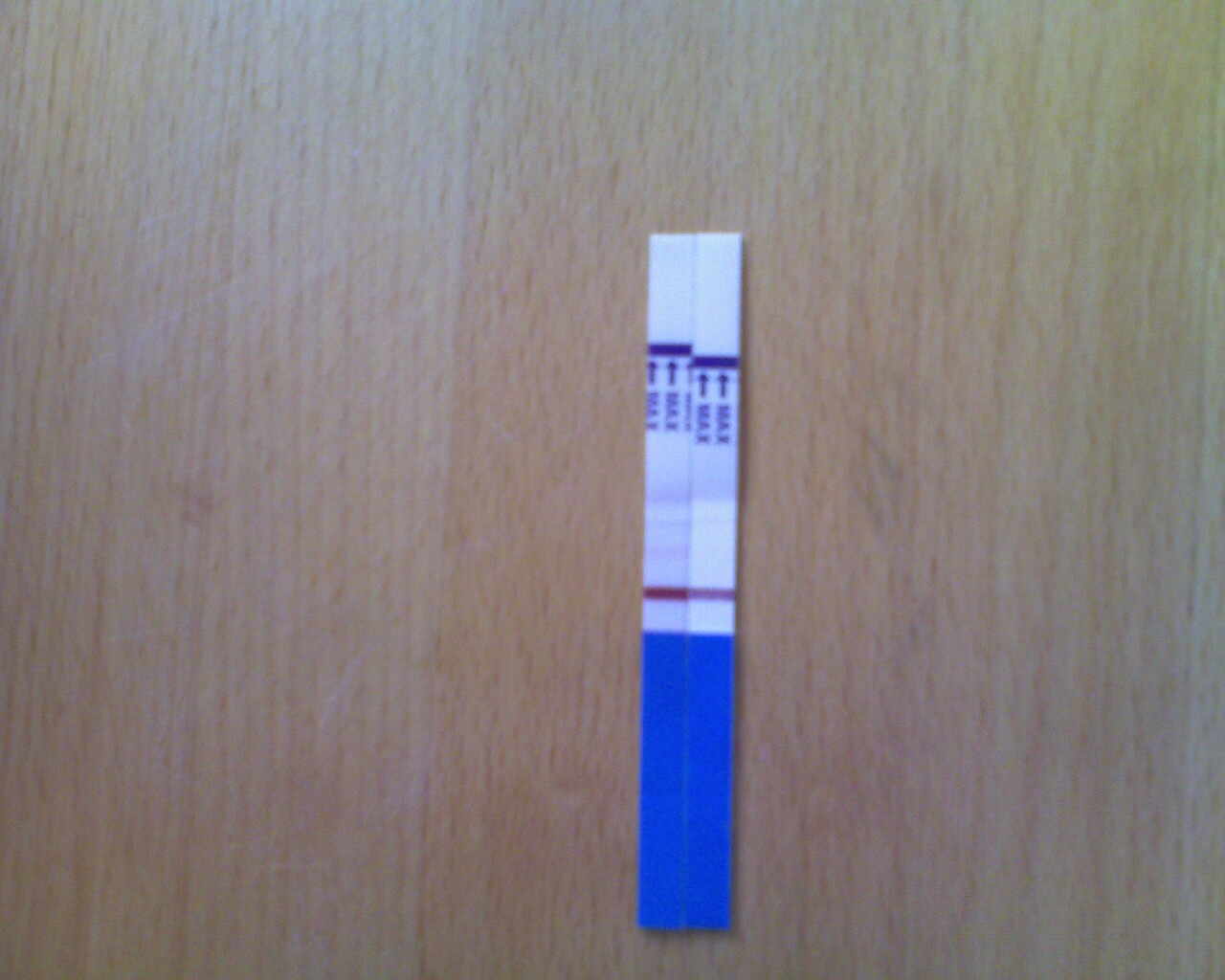A pair of test strips rest on a light-colored wooden counter or desk. Each strip features distinct color gradients: both have a blue bottom section followed by a small white segment. The first strip displays a dark purple band above the white section, while the second shows a light purple band. Just above the purple bands on each strip, the word "MAX" is printed in dark blue with a directional arrow, ending in a white tip. The specific type of test these strips are used for is unclear, but they seem to be part of a chemical testing process, possibly from a scientific laboratory environment. The desk's natural wood tones provide a neutral backdrop for the vividly colored test strips.